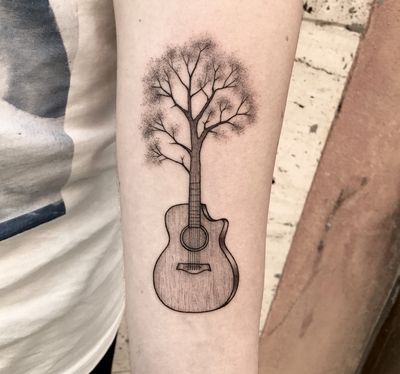The image depicts a detailed color photograph, presented in a square format, focusing on a person's forearm showcasing an intricate tattoo. The tattoo is a striking design of an acoustic guitar that transforms into a tree. The body of the guitar features a black outline with specific black outlined elements for the sound hole and the bridge where the strings would be anchored. The neck of the guitar, rendered in darker gray to resemble tree bark, seamlessly morphs into a tree halfway up, sprouting into six branches further splitting into smaller branches. These branches are fine-lined and detailed, with some ending in light gray pine needles, giving the tattoo a complex, illustrative feel. The person's skin is a light pink hue, and they are wearing a yellow t-shirt, which partially frames the image. The backdrop includes a wooden wall, with additional elements such as part of another person's white t-shirt visible on the left, adding context to the setting. This photograph showcases a blend of photographic realism and artistic representation.